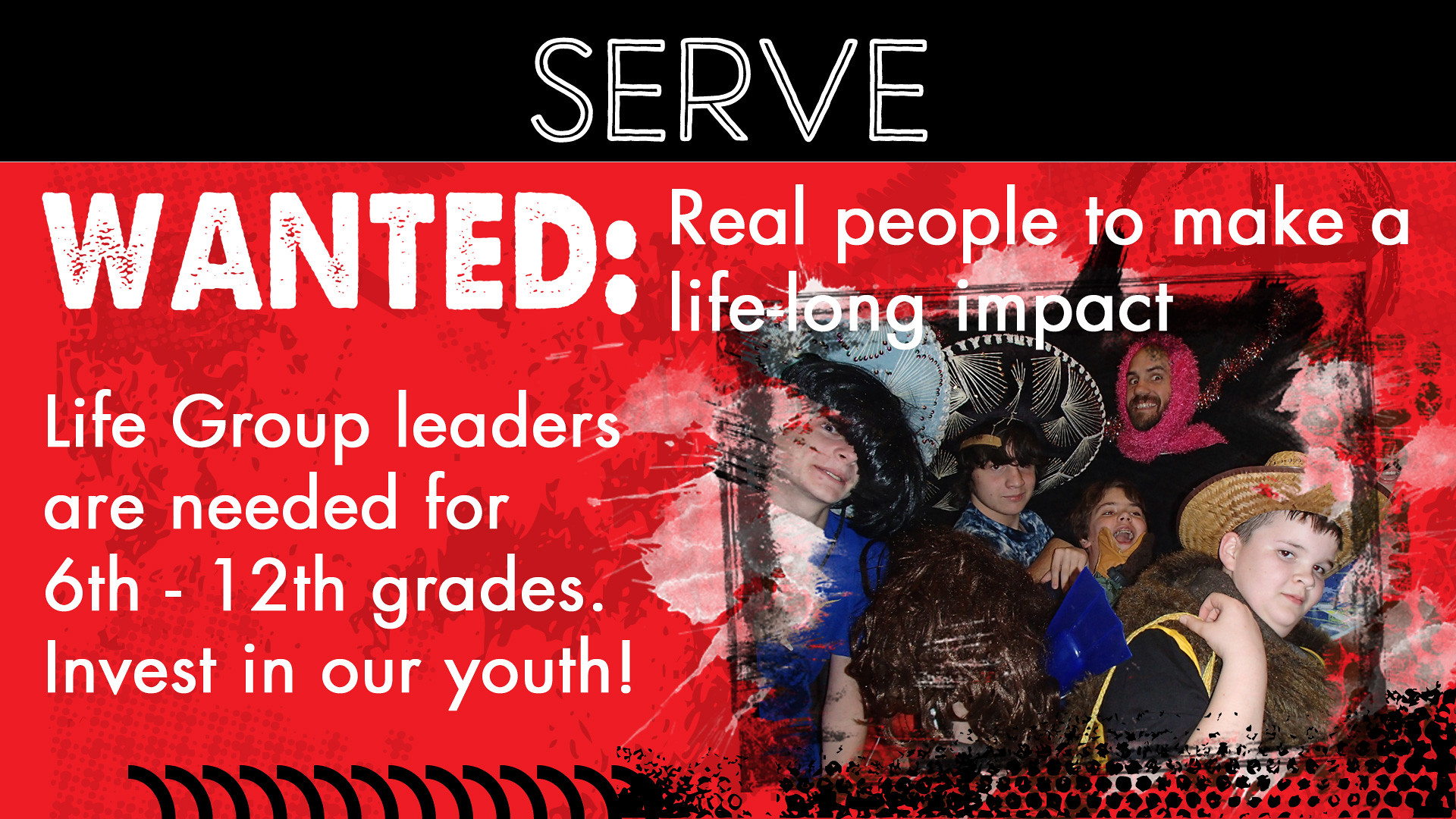At the top of the image, the word "SERVE" is prominently displayed in all capital white letters within a black border. Beneath this, a red background features bold white text that reads, "WANTED: Real people to make a lifelong impact." Below that, it continues with, "Life group leaders are needed for 6th through 12th grades. Invest in our youth." On the right side of the image, there is a lively picture of multiple boys, some wearing whimsical hats such as wicker cowboy hats and colorful Mexican sombreros. Among them is an older man with a black beard, who is playfully adorned with a feathered boa around his head and is smiling wide-eyed at the camera. The boys display a mix of expressions, ranging from serious to exaggeratedly scared, each contributing to a joyful and spirited scene. At the bottom right corner, decorative black elements, including honeycomb patterns and rows of curved lines, accentuate the overall design.